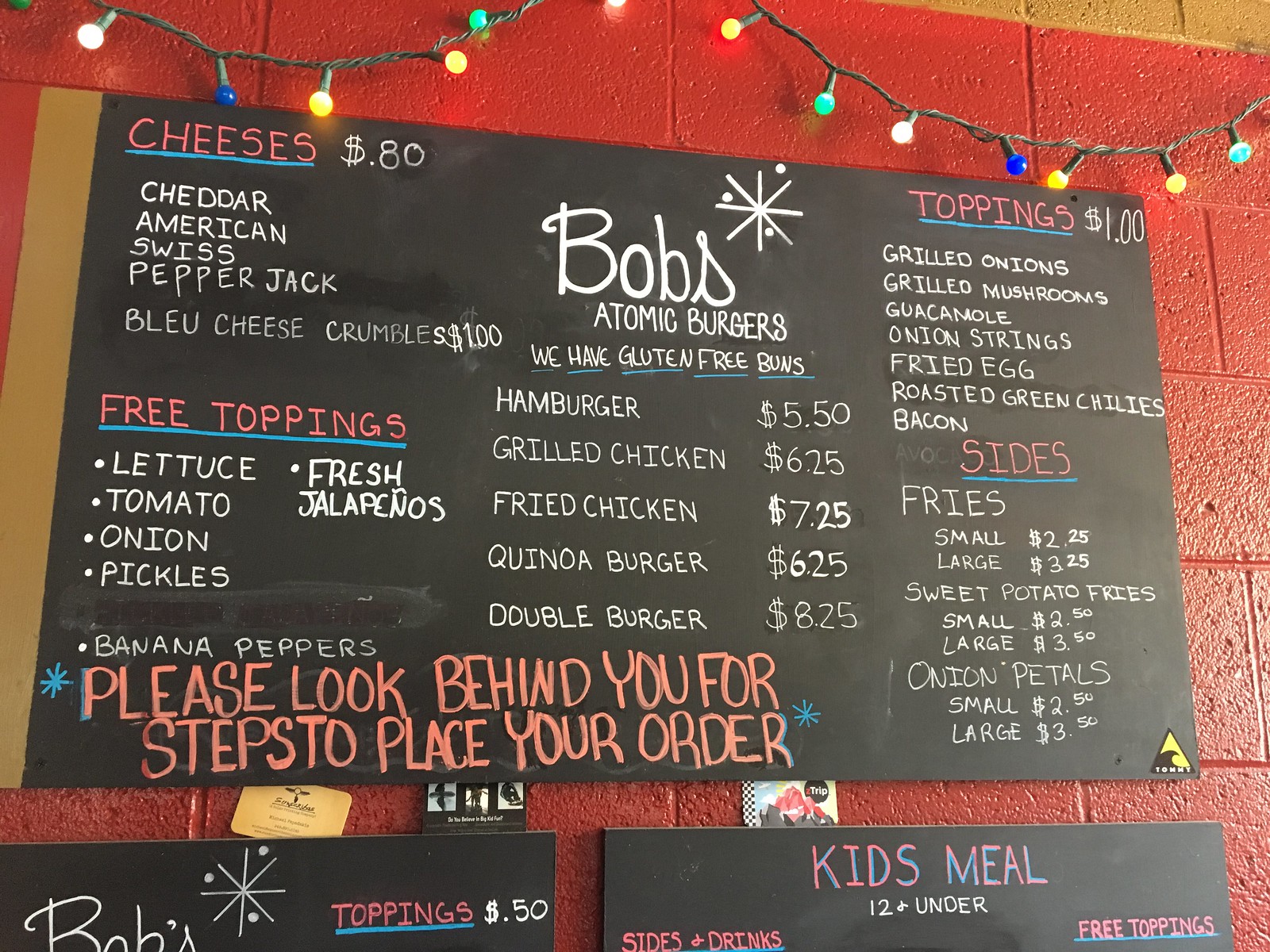In the vibrant setting of a casual eatery with a bright red wall, a large black chalkboard menu takes center stage, adorned overhead with a festive string of multicolored Christmas lights. This eclectic menu board, belonging to Bob's Atomic Burgers, features a central header with the restaurant's name artistically highlighted by a star emblem resembling an atomic symbol, evoking a playful space theme. 

The extensive menu boasts a variety of burger options including hamburgers, grilled chicken, fried chicken, quinoa burgers, and a double burger, with prices neatly listed on the side. Additional details reveal types of cheeses available for $0.80 each—Cheddar, American, Swiss, and Pepper Jack—with blue cheese crumbles available for $1.00. A list of free toppings such as lettuce, tomato, onions, pickles, fresh jalapenos, and banana peppers is provided, although it appears one topping has been erased, indicating it is temporarily unavailable. Noteworthy is an asterisk directing patrons to "please look behind you for steps to place your order," hinting at further instructions likely posted elsewhere in the establishment.

To the right of the menu, premium toppings priced at $1.00 each are listed, including grilled onions, mushrooms, guacamole, onion strings, fried onions, fried eggs, roasted green chilies, and bacon. An erasure partially obscures the word "avocado," suggesting it was also an option at one point. The menu also details side offerings such as fries, sweet potato fries, and onion petals in both small and large sizes.

Beneath the main chalkboard, two smaller menus partially visible hint at additional offerings. One mentions more toppings at $0.50 each, along with the recurring atomic symbol, while the second menu outlines a kid's meal for children 12 and under, inclusive of sides, drinks, and free toppings, though specific items remain unreadable due to the cropped photo. Adding to the casual charm, three business cards are tacked between the menus, connecting this vibrant spot to the local community.